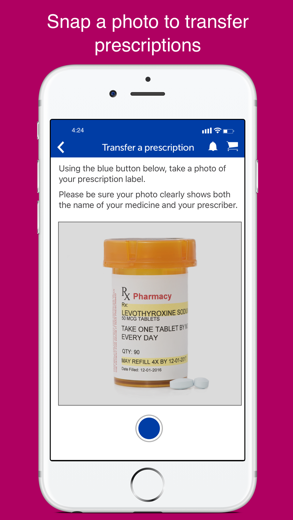This screenshot captures a streamlined tutorial from a pharmacy website on how to transfer prescriptions using an iPhone. The top of the screen features a blue banner with the text "Transfer a Prescription." Below, detailed instructions guide the user to use the blue button to take a clear photo of their prescription label, ensuring the medicine's name and prescriber information are visible.

An example prescription bottle is shown, with highlighted details emphasizing the importance of capturing the correct information. Surrounding the iPhone image showcasing the tutorial is a pink box that provides additional tips on snapping a photo for an easy and efficient prescription transfer process—all achievable with just a few clicks.

Additional icons, such as a bell for notifications and a shopping cart, indicate that this is a comprehensive pharmacy website where users can manage prescriptions and shop for new medications. The status bar also displays Wi-Fi connectivity, battery life, and the current time. The overall design predominantly uses white with blue accents for a clean and intuitive user interface.